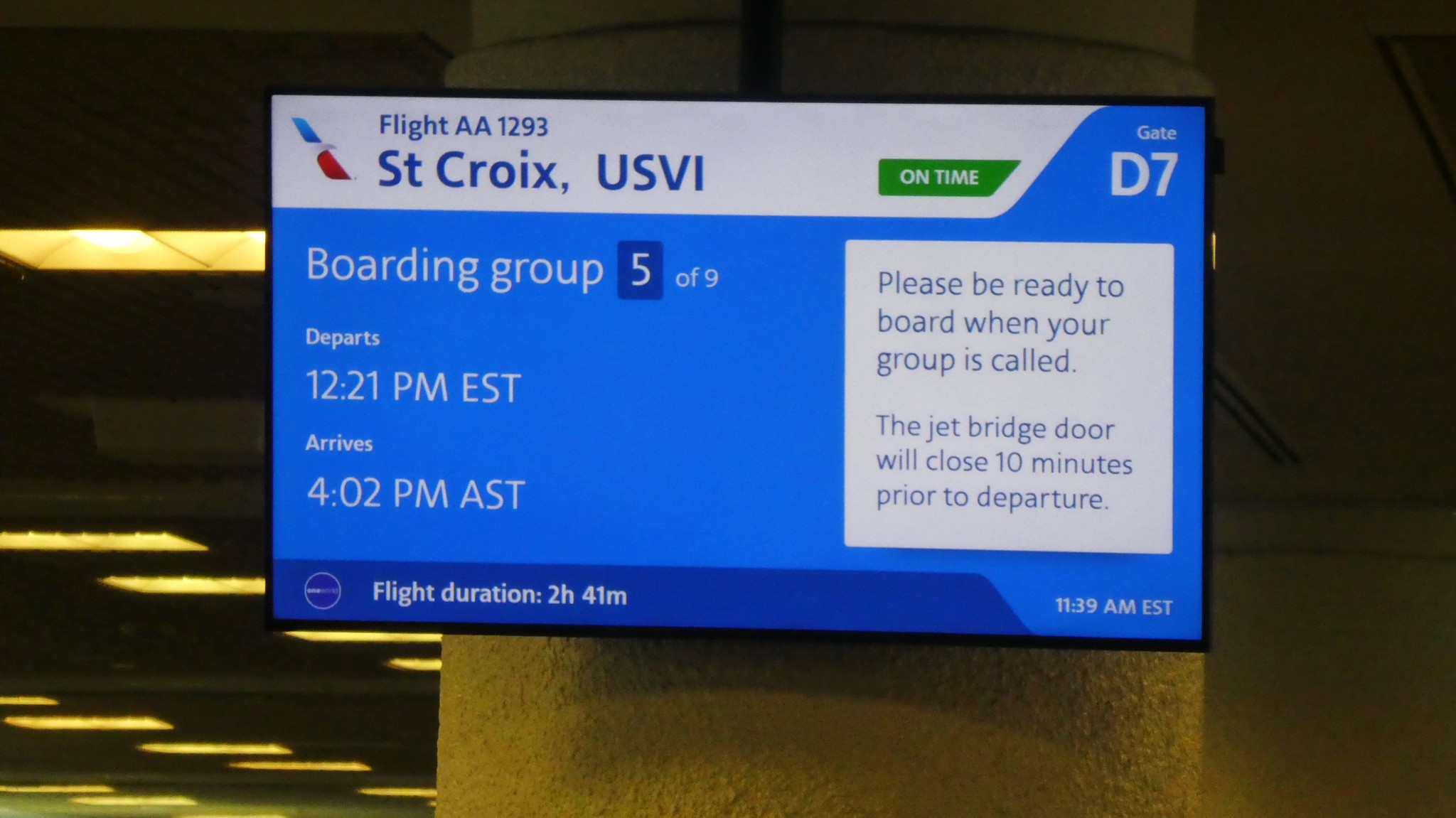The photograph captures a flat-screen television mounted on a stone column within an airport, partially surrounded by recessed yellow fluorescent lighting and what appears to be a cement parking garage in the background. The screen is predominantly blue with white, green, and red text. At the top of the screen, it displays "Flight AA1293 St. Croix USVI" in a white section, followed by a green box indicating "on time". To the right, the screen announces "gate D7". It further details, "boarding group 5 of 9" with a warning that passengers should "Please be ready to board when your group is called. The jet bridge door will close 10 minutes prior to departure." The flight departs at "12:21 p.m. EST" and arrives at "4:02 p.m. AST". At the bottom, in white font, it mentions the "flight duration is 2 hours 41 minutes" and the current time displayed in the bottom right corner is "11:39 a.m. EST".